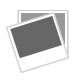The image displays a decorative cloth, resembling a poncho or large handkerchief, hanging on a brass-colored coat hanger, with the top part of the hanger visible. Primarily light brown in color, the cloth features a darker brown border along its edges. It is intricately embroidered with a variety of images, potentially depicting birds and floral prints, though the exact details are not entirely clear. There are approximately six different types of birds, including a swan, a purple bird, and a yellow flying bird, nestled amongst floral patterns on the main lighter section of the cloth. The cloth is neatly folded over the hanger, with three pointed sections at the bottom, and is set against a plain white background, giving a clear perspective of its design and size.